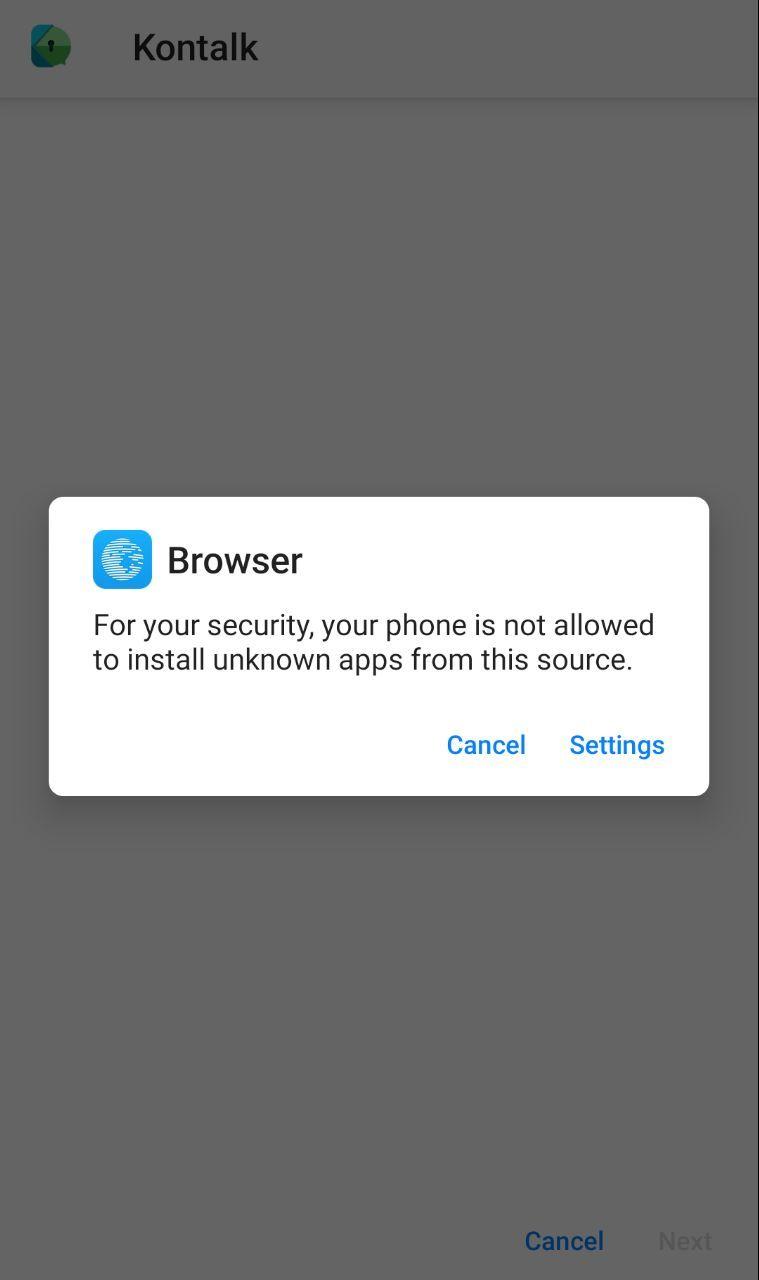The image appears to be a screenshot taken from a smartphone, but it does not include the status bar that typically shows the time and signal strength. At the top left corner, there is the word "KONTALK" with a corresponding icon next to it. The background of the screenshot has a shadowed, light gray appearance. Below the "KONTALK" section, a white overlay box displays a security warning message: "For your security, your phone is not allowed to install unknown apps from this source." Below this message, options to "Cancel" (highlighted in blue) and "Settings" (also in blue font) are presented. Additionally, at the very bottom of the screen, there are two more buttons labeled "Cancel" and "Next," with the "Cancel" button's text also in blue. Inside the white overlay box, there is an icon resembling a rounded rectangle with a globe symbol inside, indicating an internet-related function.